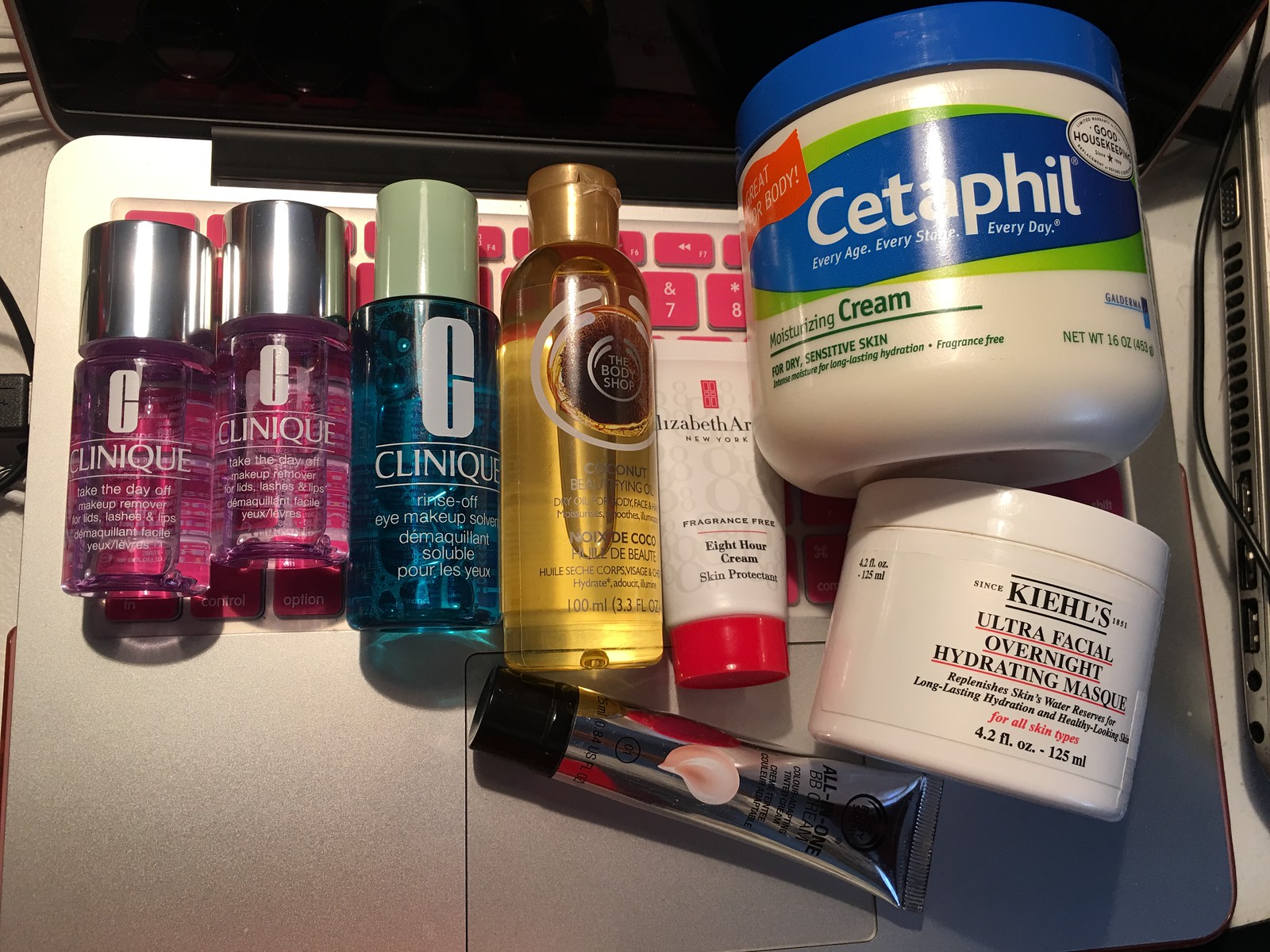In this image, a variety of beauty products are artfully arranged on top of an open silver laptop with distinctive pink keys. Starting from the left, there are two clear bottles filled with pink liquid. Both bottles feature the recognizable "C" logo of Clinique and have silver caps. Adjacent to these, a clear bottle containing teal-colored liquid also from Clinique can be observed. This product is labeled as an eye makeup removing serum and is topped with a green lid.

To the right of the Clinique items, there is a gold bottle showcasing the brand name "The Body Shop." Next in line is a tube of Elizabeth Arden's Eight Hour Cream, renowned for its multi-use skin benefits. Following this, a larger container of Cetaphil lotion can be seen, easily identifiable by its blue accent and green stripe. 

Below these items lies a jar of Kiehl's Ultra Facial Overnight Hydrating Mask, clearly marked as containing 4.2 fluid ounces. Finally, at the bottom of the arrangement, there is a silver tube with a black cap, possibly containing makeup or lotion.

The laptop beneath these beauty essentials adds an additional layer of interest to the composition, with its black screen situated at the top of the image and pink number keys '7' and '8' prominently featured.